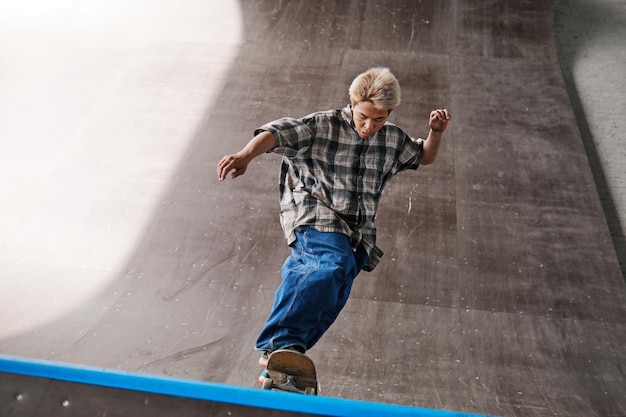The photograph depicts a young skateboarder with dyed blonde hair, wearing an oversized plaid shirt and baggy blue jeans. He is on a steep, gray skateboard ramp that has visible marks and a blue strip edging at the top. The skateboarder appears to be concentrating on maintaining his balance as he maneuvers the ramp, glancing downwards at his skateboard. Sunlight illuminates the left side of the image, casting a contrasting shade over the right side. His arms are extended outward to aid his balance as he navigates the incline of the ramp.